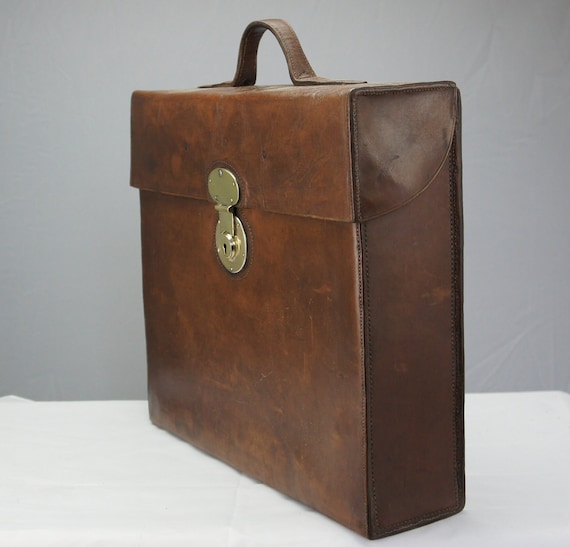The image is a color photograph in a square format, depicting a brown leather briefcase standing upright on a white table covered with a slightly wrinkled white tablecloth. The briefcase is angled so that both the front and the right side are visible. The leather is a dark reddish-brown with various scratches and imperfections, while the front flap is a slightly lighter, warmer-toned brown. The handle at the top is made from the same dusky brown leather. The closure is a brass clasp with a circular design and a keyhole, centered on the front flap. The background consists of a light gray wall, with some fabric wrinkles visible on the right side of the image. The overall style of the photograph is realistic, highlighting the texture and details of the briefcase in a product photography setting.